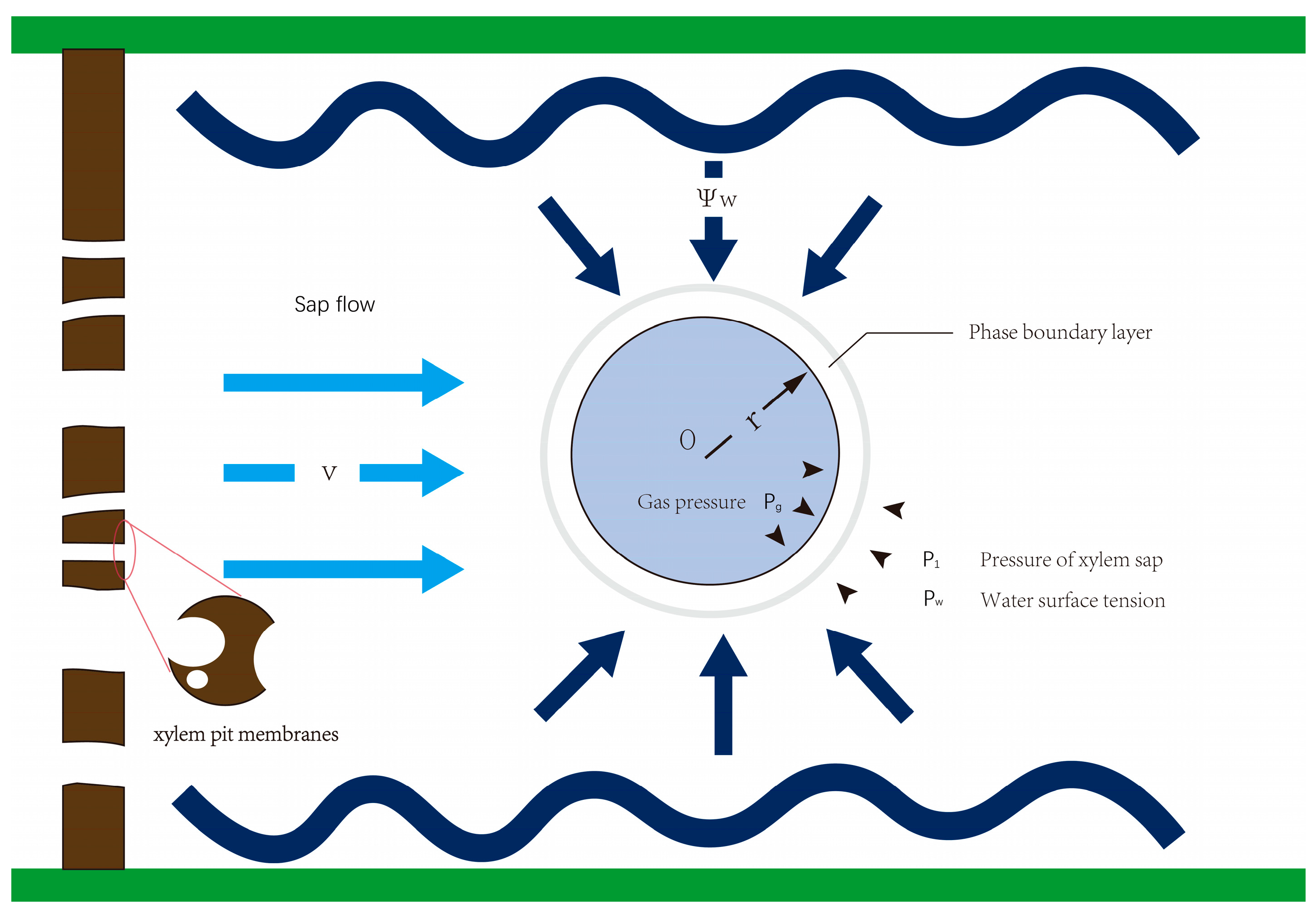This infographic, depicted in a simple, almost cartoonish style, illustrates the function of a xylem pit membrane. Dominated by various shades of blue with accents of green and brown, the diagram features a prominent brown vertical line on the left side indicating the xylem pit membranes, with segments missing, suggestive of microscopic holes. The top and bottom sections are highlighted by green horizontal lines functioning as a header and footer. Dark blue squiggly lines extend from these green lines, with arrows pointing towards and within a central blue circle. Annotations within and around the circle detail key concepts such as "sap flow," "boundary pressure layer," "pressure of xylem sap," "water surface tension," and "gas pressure." The circle itself contains symbols and letters, including 'R' for radius, 'P' for pressure, and 'O' for oxygen, alongside mathematical notations, visually representing the internal mechanics of gas pressure within the pit membrane. This diagram is likely intended for educational purposes in a science course, specifically to elucidate the dynamics of xylem sap flow and related pressures.